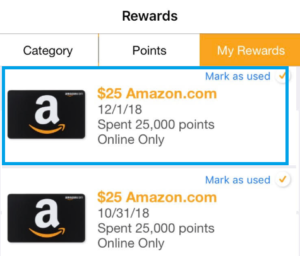This is a cropped image of a screen from what appears to be the mobile app or mobile website of Amazon. The interface is primarily displayed on a white background. At the top center in black text, the word "Rewards" is prominently visible. Below this heading are three buttons: "Category" and "Points" on the left, both in white, and "My Rewards" on the right, highlighted in orange. 

Beneath these buttons is a large blue box that outlines one of the rewards listed. Both rewards depicted feature an image resembling an Amazon credit card, characterized by a black background, the Amazon logo with its iconic smile arrow, and a lowercase sans serif "A" in the middle.

The highlighted reward card shows orange text indicating "$25 Amazon.com," accompanied by the date "12-1-18." It specifies that 25,000 points were spent, and this reward is marked for online use only. The reward card below it, which is not highlighted, is nearly identical but shows a different date, "10-31-18."

Both reward entries include white radio-style checkmarks with orange checkmarks inside them, next to blue text that reads "Mark as used." The blue box's slightly off-center appearance suggests it is being used for demonstration purposes rather than being a part of the actual user interface, likely to draw attention to the highlighted reward.